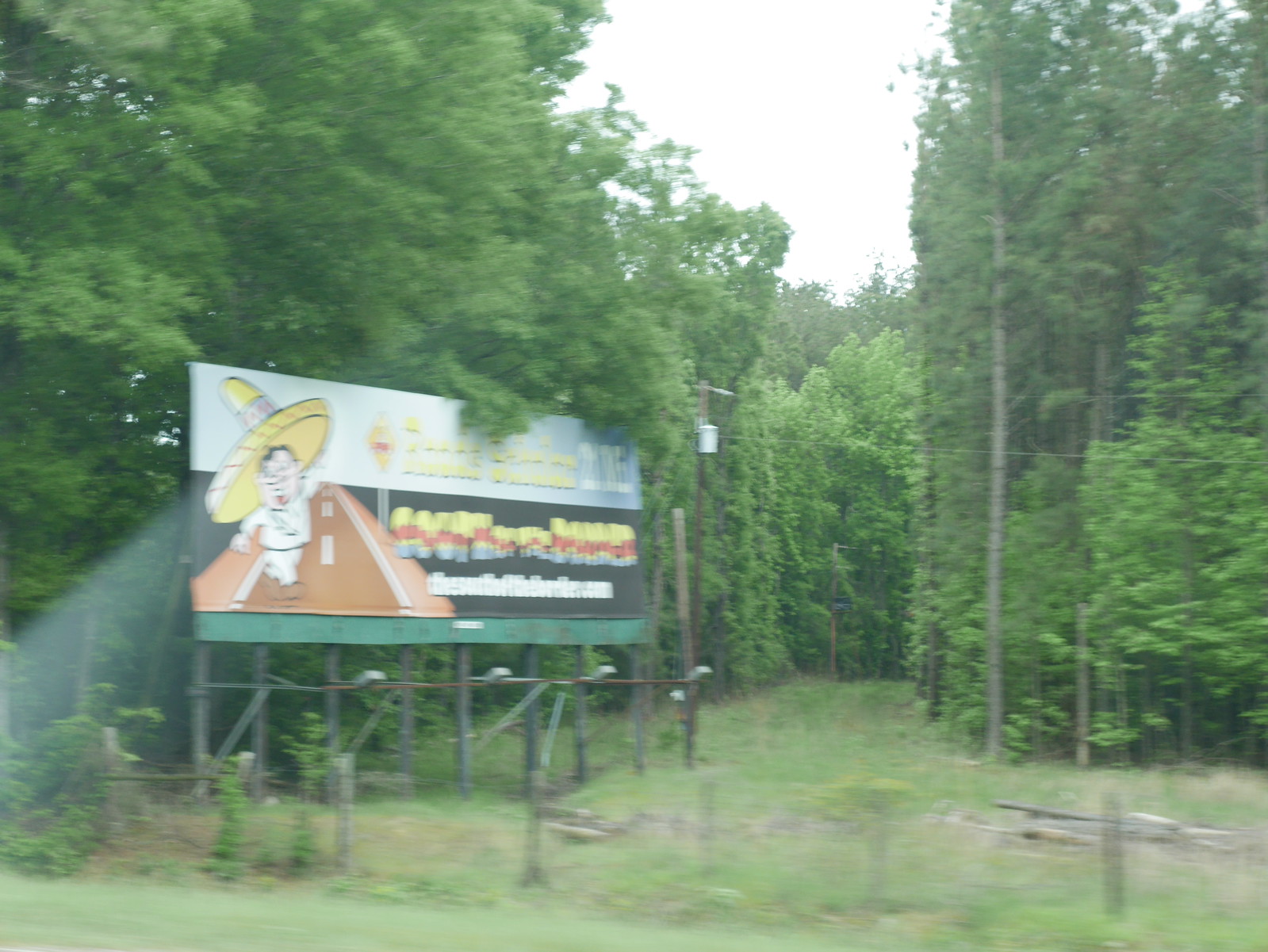The blurry color photograph depicts a rural scene dominated by a billboard, positioned amidst a densely wooded area just south of the North Carolina-South Carolina border. The billboard, intended to attract tourists to a tacky attraction called "South of the Border," features a cartoon image of a man in a large yellow sombrero dancing down an orange road. The background of the billboard is split into a blue upper half and a black lower half, with the words "South of the Border" visible along with a website, although portions of the text remain illegible due to the blur. The area surrounding the billboard consists of a mix of pines and hardwoods, interspersed with grass and a clear path that includes utility lines adorned with a transformer. The foreground shows low fencing made from two-foot posts possibly linked by chicken wire, depicting a rural landscape through which the road cuts. The photograph appears to be taken from a moving car, adding to the overall impression of motion and the day's journey.